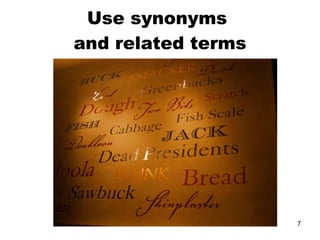This image, found on Prolific, features a collection of words displayed in various fonts and colors, primarily black and red. At the top, the phrase "Use synonyms and related terms" is prominently displayed. Below this directive, the image showcases an array of words, each styled uniquely—some in capital letters, others in lowercase, with a mix of regular print, Times New Roman, cursive, and other decorative fonts. The words include terms such as "dough," "cabbage," "fish scale," "jack," "dead presidents," "bread," "sawbuck," "shrimp," "shrimp blaster," "fish," and "buck," among others.

Each word is depicted in either black or red ink, creating a stark visual contrast. Some words have intricate details; for instance, the word "dead president" features a partial light reflection, illuminating the letter 'P'. The background of the image has a warm, earthy palette, combining shades of brown, yellow, and cream, which provides a muted yet complementary backdrop for the vivid text.